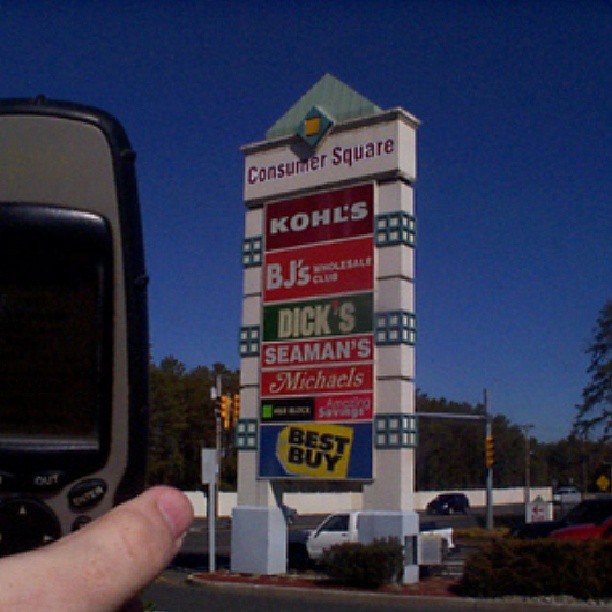The image features a tall, prominent billboard against a clear blue sky, situated at a location known as "Consumer Square." The text on the billboard lists several store names in descending order: Kohl's, BJ's, Kohl's Hill, Dick's, Seaman's, Michael's, H&R Block, and another partially obscured store sign. At the bottom, a visible sign for Best is also displayed. A finger, presumably that of the person taking the photo, points ambiguously toward the sign. The photograph is captured during the daytime, with large trees visible in the background. Additionally, the reflection of a vehicle’s passenger-side mirror suggests the photo was taken from inside a car.